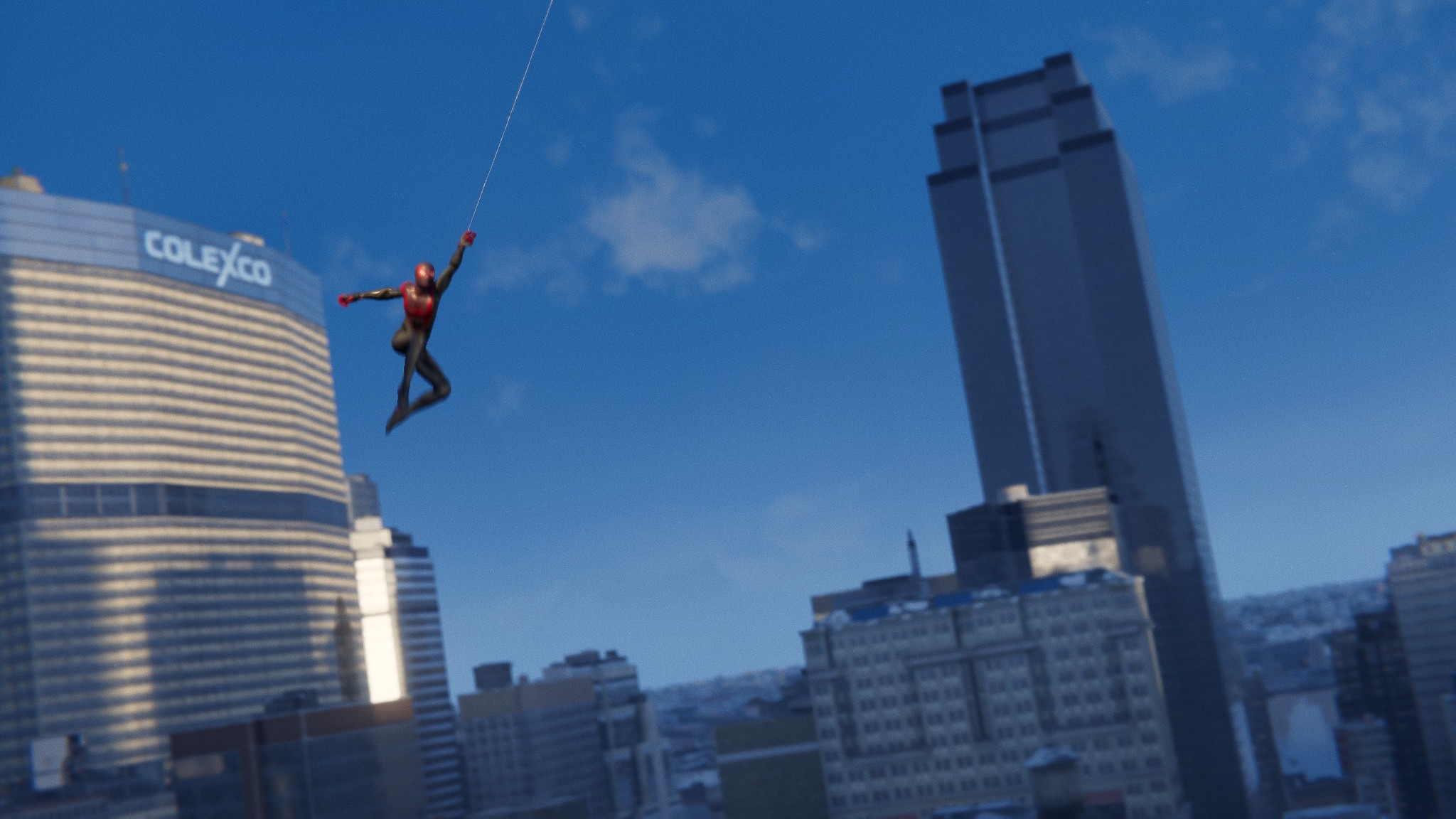In this dynamic image, a superhero resembling Spider-Man is captured mid-swing, connected by a web or string to an off-frame point at the top of the picture. The hero, clad in a striking black tightsuit accented with a red helmet, red chest plate, and red gloves, appears to be in the midst of downtown skyscrapers. The buildings, including one prominently labelled "Colexco," are set at a slight angle, suggesting the photo was taken from an unconventional perspective. Against a backdrop of a vivid blue sky adorned with fluffy white clouds, the scene conveys a sense of height and motion. Additional structures, possibly smaller buildings or houses, can be seen in the distant background, further emphasizing the urban setting. The superhero is swinging dynamically from the left side to the right side of the frame, adding an exhilarating sense of action and adventure to the visual narrative.